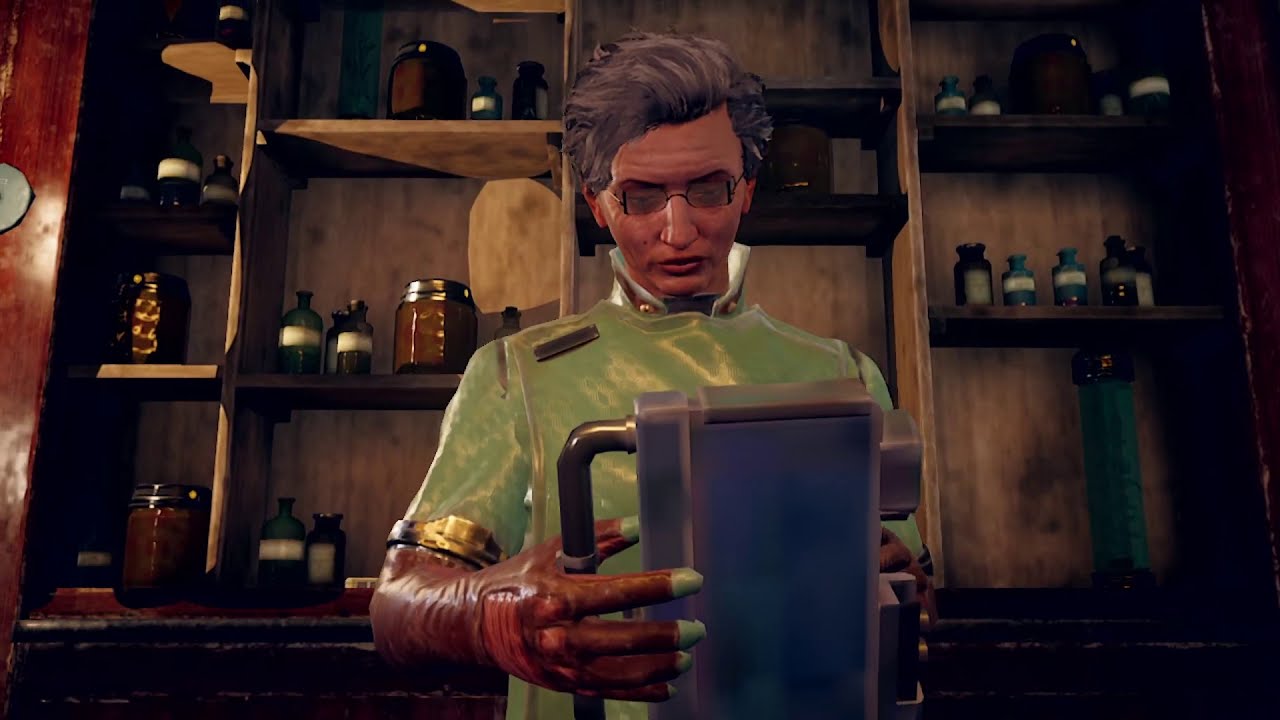The image depicts a detailed, 3D-rendered character from a video game, likely rendered with PlayStation 4 quality graphics. The character appears to be male, with short gray hair, light reddish skin, and small sunglasses. He is wearing a minty green short-sleeve jacket with gold trim on the sleeves and long brown, wrinkly gloves that might be part of a protective uniform. He stands facing away, looking intently at a metallic blue item with a handle, which he holds in his hands. The background is a wooden shelf unit adorned with various glass jars and bottles with labels, some with gold lids, others black and beige, creating a dense and meticulous arrangement. The overall scene suggests a setting in a laboratory or apothecary, with a significant emphasis on the well-detailed environment, enhancing the immersive experience of the game.